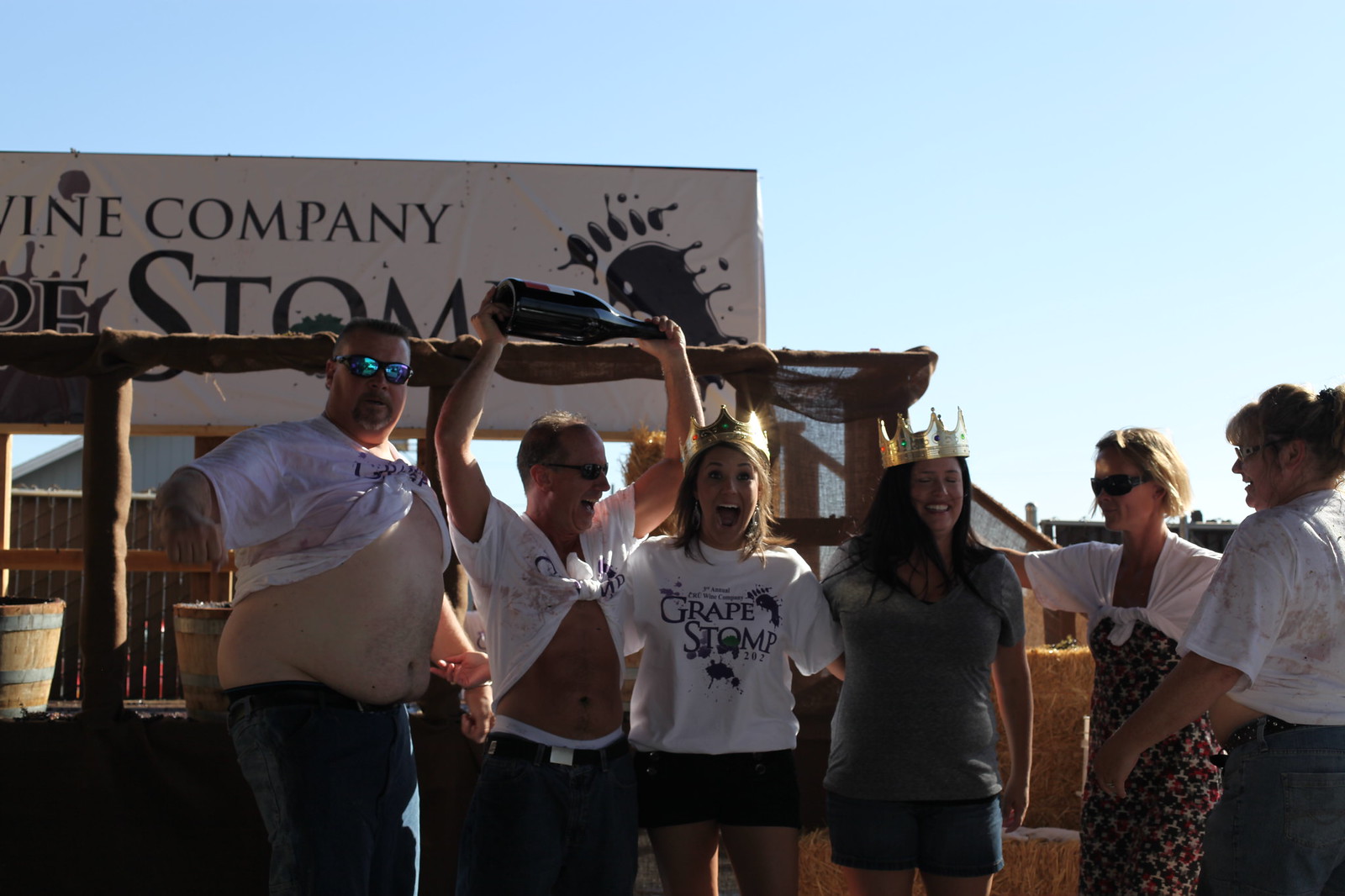In this horizontally aligned rectangular picture, a group of six people stands at an outdoor event under a clear blue sky. A large sign to the left partially reads "company" and "stomp," along with a splattered footprint, indicating a grape stomp event. 

Starting from the left, a man with a large belly, revealed by his lifted shirt, poses in black pants and sunglasses, staring directly at the camera with a confident stance and short brown hair. Next to him, another man displays his stomach with his shirt tied up on his chest, holding a large wine bottle above his head, laughing, and also wearing sunglasses. 

In the middle stands a woman with short blonde hair, a golden crown, and an open-mouth smile, dressed in a white "grape stomp" T-shirt with splattered footprints and black shorts. Adjacent to her, another woman in a gray T-shirt with blue jean shorts and long brown hair smiles broadly with her eyes closed, also wearing a gold crown.

On the far right, two women appear to be presenting a winning reward to the group. One has short blonde hair and wears a brown dress with a white top and sunglasses, while the other, partially visible, sports a white T-shirt turned sideways. 

In the background, bales of hay and grape stomping buckets on a platform enhance the festive atmosphere of this grape-stomping event.